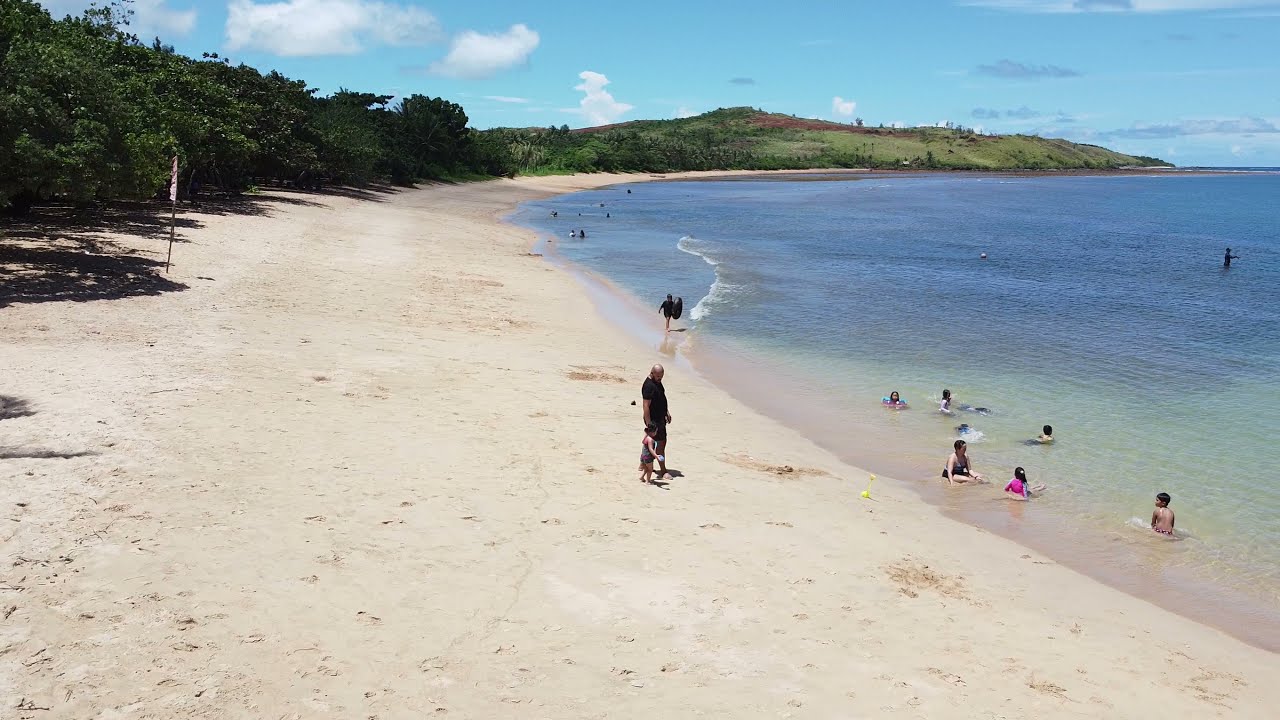This outdoor daytime photograph captures a picturesque beach scene with a lengthy sandy shoreline curving along the right side and wrapping back toward the left. The sand starts at the bottom corners of the image, with the shore forming a semicircle as it narrows toward the deeper bluish-green ocean. The water transitions from a lighter brownish-green hue in the foreground to a deeper blue farther out.

In the foreground, a tall, bald man dressed in a black shirt and shorts holds the hand of a very young girl facing the sea. To the right, there are nine people, mostly children, some playing in the shallow water and others sitting in the sand. One woman, distinct in a black one-piece bathing suit, stands among them. 

A lush stretch of vegetation, including trees and grasses, lines the left side of the sand. In the distance, a green mountain topped with what seem to be white houses stretches across the backdrop. Above, the bright blue sky transitions from fluffy white clouds on the left to darker gray clouds on the right, adding depth and contrast to the tranquil beach setting.